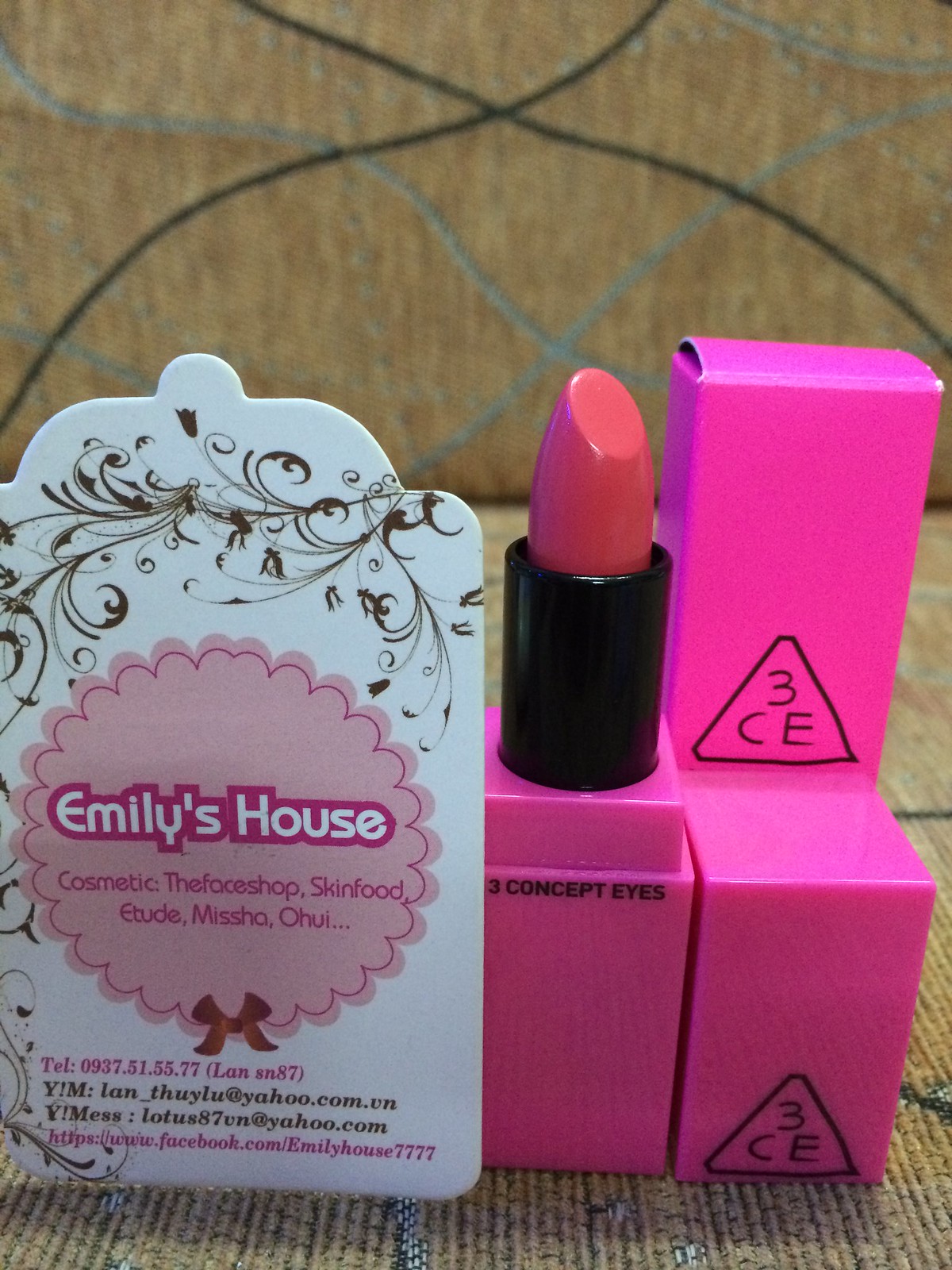The image shows an arrangement of beauty products on a light brown surface, likely a couch or chair, with wavy gray and black stripes. On the left side, there is a white plastic piece with a pink cloud-like design in the middle, displaying various beauty brand names such as "Emily's House Cosmetic, The Face Shop, Skin Food, Etude, Missha, Ohui." Below this, there is a detailed text that includes a contact number (0937.51.55.77), an email address (yimlanthuly@yahoo.com.vn), and a Facebook URL (https://www.facebook.com/EmilyHouse7777). To the right, an open reddish-pink lipstick with a glossy black tube is placed on top of one of three pink boxes, all with a black triangular "3CE" logo, indicating the brand "Three Concept Eyes." The background is the same light brown, with the bottom of the box mirroring the light brown and tan hues. The overall scene appears compact yet detailed, showcasing specific cosmetic brands and contact information amidst a cozy setting.